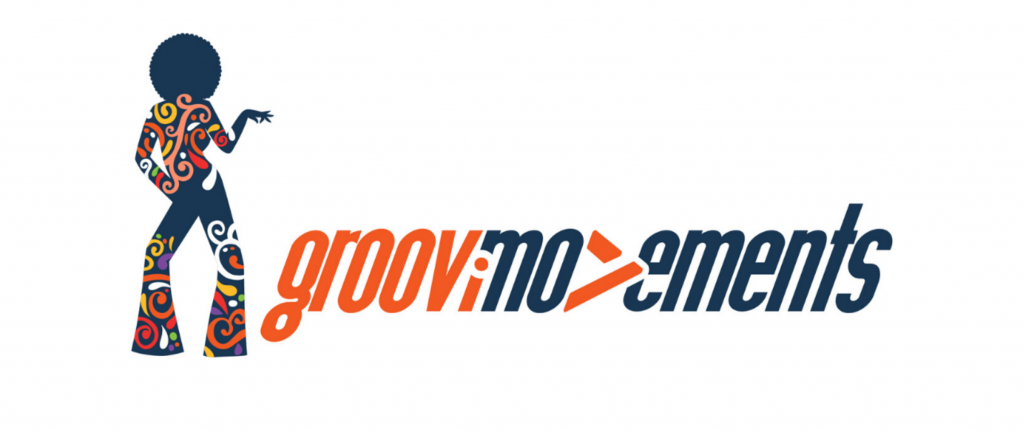This digital, computer-generated image depicts a logo and brand name on a white background. On the left side, there is an outline illustration of a person in the midst of a dance pose, turned slightly with their back facing outward. The person has an afro and flared pants, with one arm extended to the side forming a sign with their hand and the other hand resting on their hip. The figure showcases a vibrant, colorful design on their torso and legs, featuring shades of orange, yellow, red, green, pink, and white against a predominantly blue outline. On the right side of the logo, the brand name "GROOVMOEMENTS" is presented in a stylish font. The first part of the name, "GROOV," is colored orange, while the latter part, "MOEMENTS," is in blue, with a distinctive orange triangular shape introduced between the ‘O’ and ‘E.’